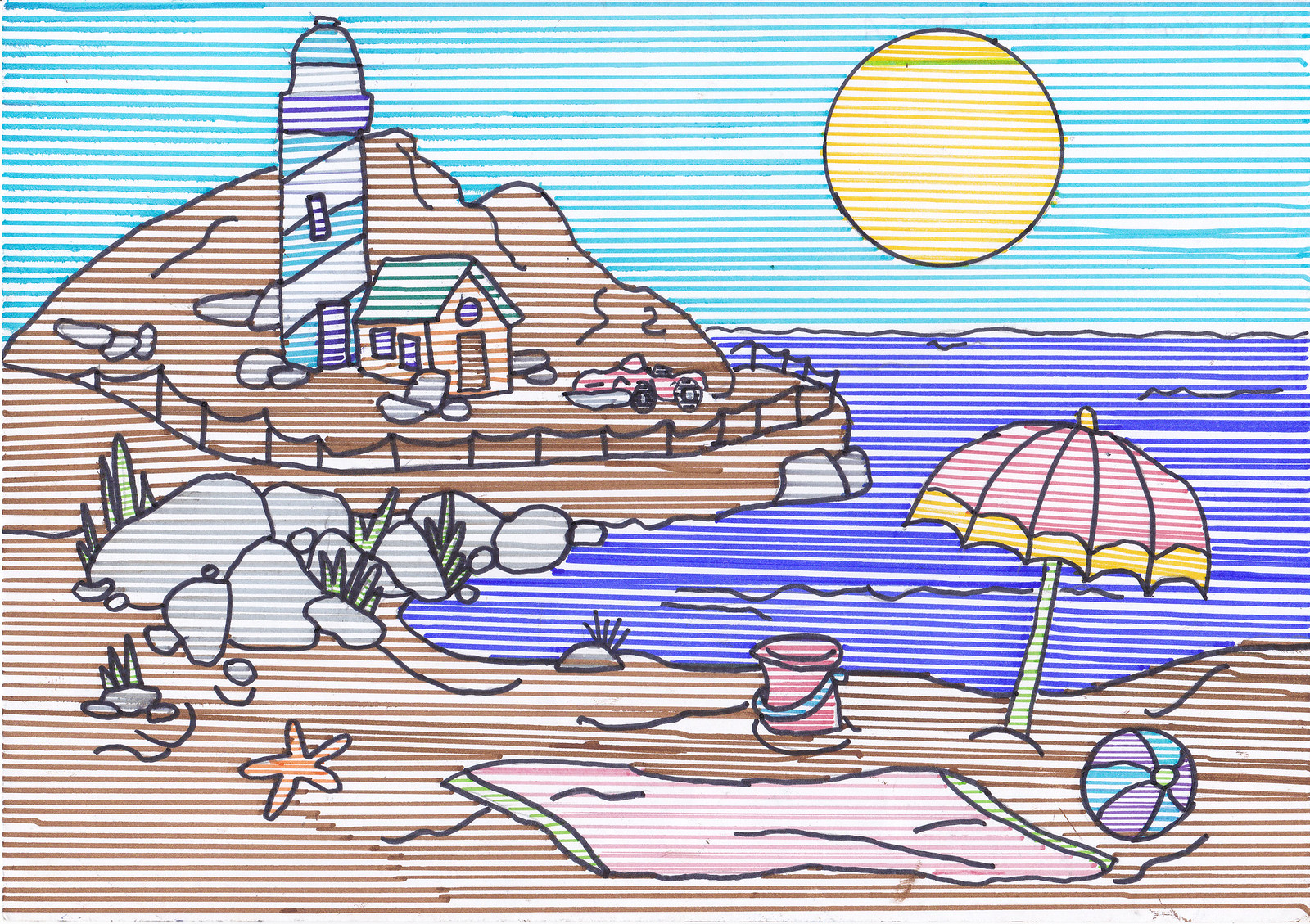This image is a detailed line drawing that appears sketched using colored pencils. The top half of the image features a light blue sky filled with thin horizontal lines. Towards the top right, a yellow sun, outlined in black, radiates with delicate horizontal yellow lines. Below the sky on the left, there are brown mountains with finely shaded brown lines, topped with a green-roofed, brown house. The house includes a purple round window, two smaller windows with black outlines, a little brown door with a black outline, and a tower adorned with vertical turquoise and gray stripes. A red sports car with black wheels is parked in front of the house.

The middle section of the drawing transitions from the mountainous terrain to a dark blue ocean, represented with similar thin lines. Surrounding the island where the house and lighthouse stand, rocks delineated with gray hues and sparse green weeds are scattered around. 

The bottom half immerses us in a beach scene. A sandy shore, textured with thin lines, is detailed with various beach items: an orange starfish, a pink-outlined beach towel, a red pail with a blue handle, a green-yellow-red umbrella, and a multicolored beach ball. This area is adjacent to the water, edged with additional rocks and minimal green vegetation, showcasing the meticulous nature of the sketched lines throughout the drawing.